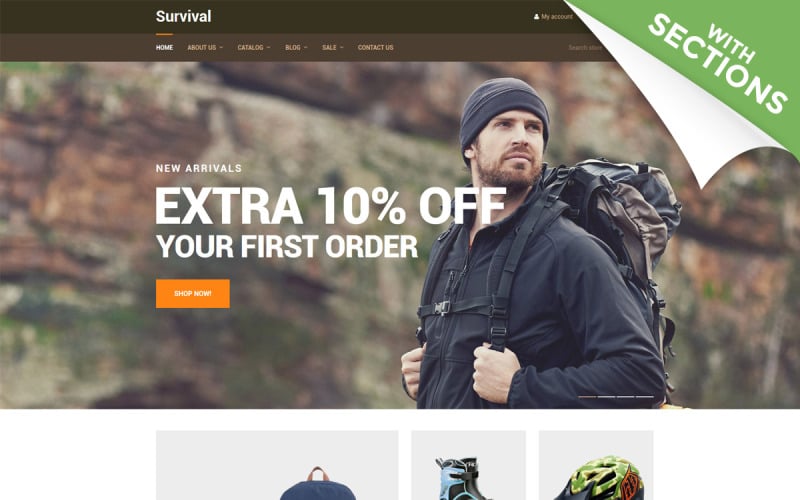The website caters to adventurers and explorers, offering an immersive and rugged design theme. At the top, a black navigation bar labeled "Survival" features a few options: "My Account" on the left and a unique turn-down effect on the right corner, revealing a green background with angled selections inviting further exploration.

Below the black bar is a brown navigation strip that includes links to "Home," "About Us," "Catalog," "Sale," and "Contact Us." Below this bar, there's a striking image of a bearded man in a toboggan hat, wearing a stylish jacket and carrying a large backpack. He stands in front of a stone wall and gazes into the distance with a visionary look.

The text on the image promotes new arrivals with a small-font announcement, and an enticing offer of "Extra 10% Off" in bold, large font. The phrase "Your First Order" follows in a slightly smaller yet bold font, all in white. At the bottom of the image, a noticeable button encourages users to "Shop Now" to take advantage of the 10% discount on their first purchase.